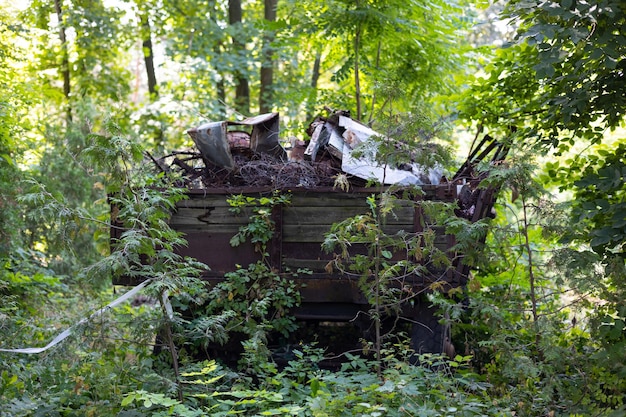In the midst of a dense, vibrant forest teeming with greenery, an old, abandoned wooden structure lies in a state of disrepair and decay. This structure, resembling the base of a conestoga wagon or an old wooden ship, is partially held together with rusted metal strips. It's topped with what appears to be a white object, now nearly obscured by thick vines and overgrown foliage, indicating it has been left untouched for a significant period. The wood is cracked and weathered, with some parts on the brink of collapse, threatening to spill the assortment of metal pieces, branches, and garbage inside. A single wheel with a tire and hub is visible at the bottom right corner, further hinting at its past life as a cart or wagon. The setting is bathed in a soft, diffused light filtering through the dense canopy of leaves, accentuating the vibrant summer greens around the forsaken relic.